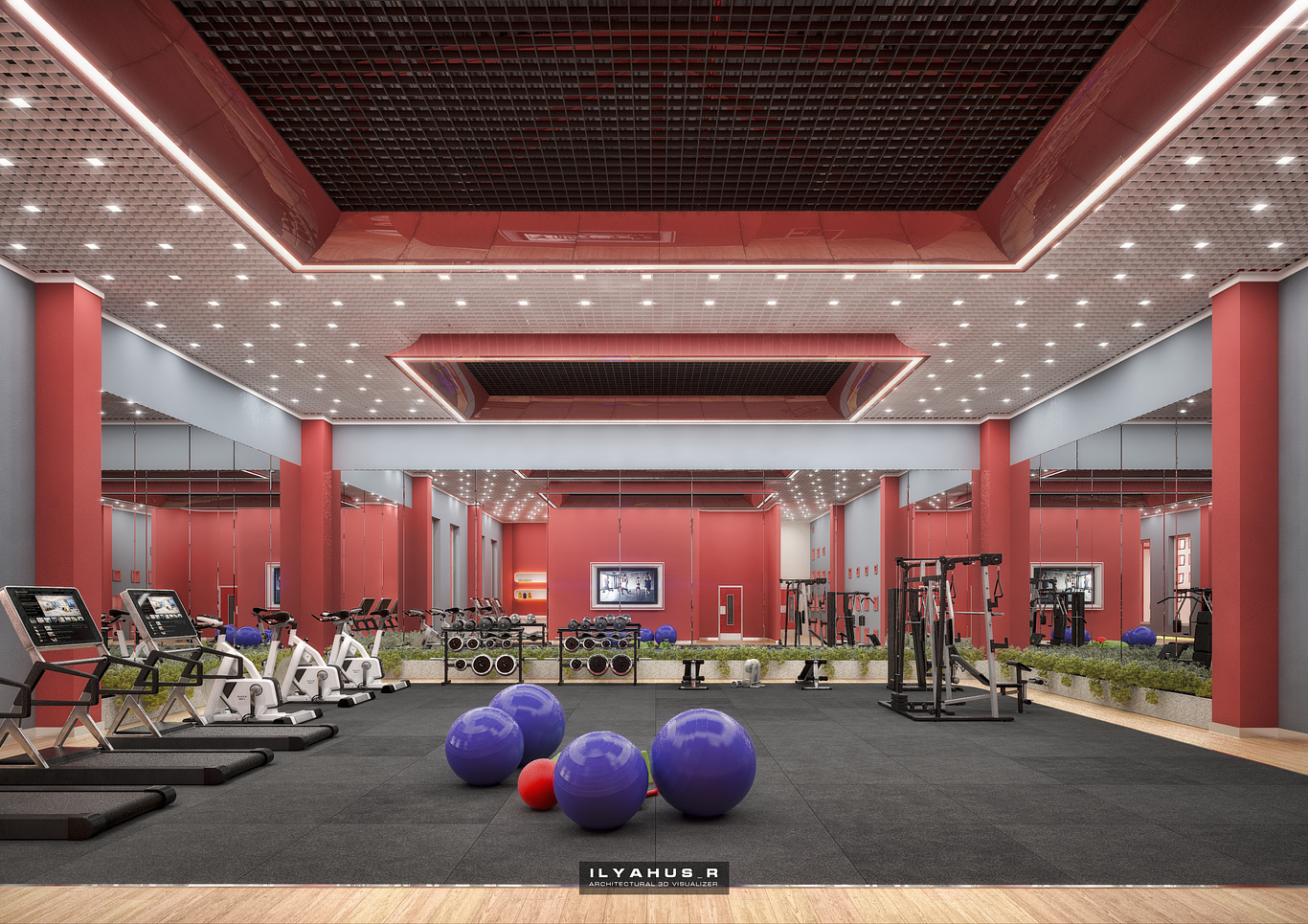The image showcases an opulent, photorealistic interior of a gym, seemingly within a hotel or conference center, identifiable by its grand, open design. The gym's flooring is composed of large gray carpet tiles, providing a sturdy base for various equipment, including a central arrangement of four purple pilates balls and one red ball on a wide black mat. To the left, a set of three treadmills is prominently positioned, adjacent to a series of white stationary bicycles. Toward the right, additional exercise machines and a Smith machine are visible, along with racks of free weights in the back.

The environment is defined by its expansive grid-style ceiling, embellished with numerous lights and an overhead structure suggestive of extensive air conditioning works. Red, brick-like columns punctuate the space, adding a vivid contrast against the mirrored walls that enhance the room's sense of scale. Low concrete planters with lush greenery border the workout area, underscoring the sophisticated and serene ambiance. 

Across the bottom of the photograph, the text "ILYAHUS." in white font is subtly placed over a black box, adding a touch of branding to the meticulously designed fitness area.